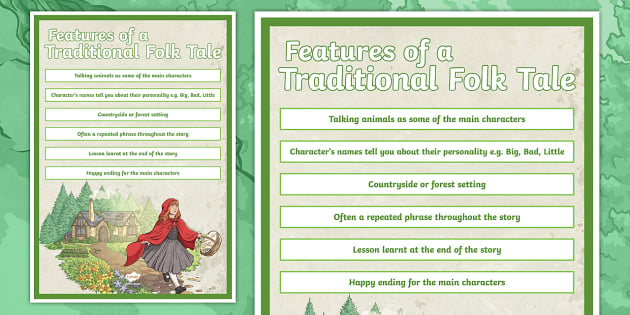The image depicts a detailed guide on the features of traditional folktales. It is presented in a format that resembles either a PowerPoint slide or a flyer. The guide is divided into two sections: the left side shows a full-page view, while the right side features a zoomed-in portion focusing solely on the text. The headline, "Features of a Traditional Folktale," is prominently displayed in white text with a green outline.

Beneath the headline, there are six text boxes outlined in green and filled with details in white rectangles, containing green text. These boxes list the defining characteristics of traditional folktales: talking animals as some of the main characters; characters' names that reveal aspects of their personalities (e.g., "Big Bad" or "Little"); a countryside or forest setting; the frequent repetition of certain phrases throughout the story; a lesson learned either during or by the end of the story; and a happy ending for the main characters.

Additionally, the left side includes an illustration of Little Red Riding Hood walking down a path, holding a basket, and wearing her iconic red cape and hood. In the background, there is a house situated within a forest, evoking the classic folktale setting.